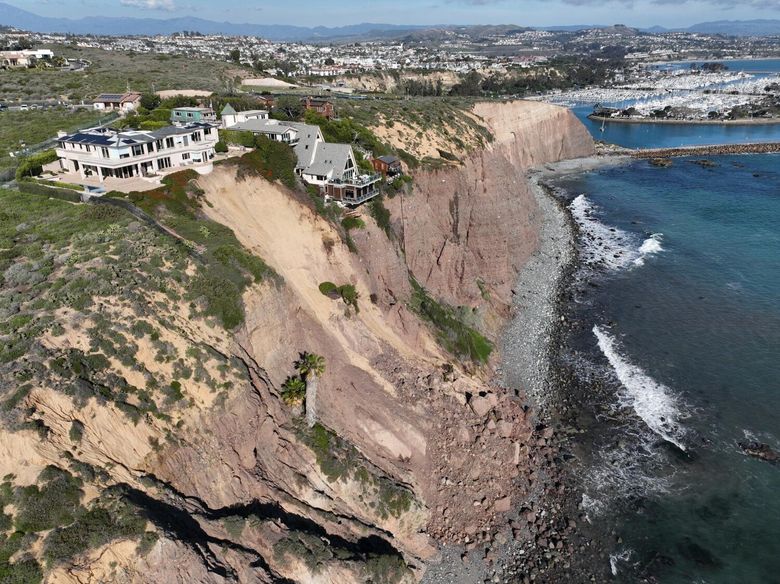An aerial photograph captures a dramatic cliffside landscape bathed in sunlight, where luxurious mansion houses perch perilously close to the edge. The cliff shows visible signs of erosion with its layered shards of rock in various shades of browns and tans. Sparse greenery dots the sandy terrain, enhancing the rugged beauty of the scene. Below, the rocky coastline meets the aquamarine water with waves cresting and white bubbles forming at the surface. The background reveals a picturesque horizon with additional houses, expansive mountains, and a clear, light-colored sky, hinting at a serene yet precarious coexistence of nature and human habitation. To the top right, a peninsula extends into the water, adorned with more residences, enhancing the complexity and richness of the vista.